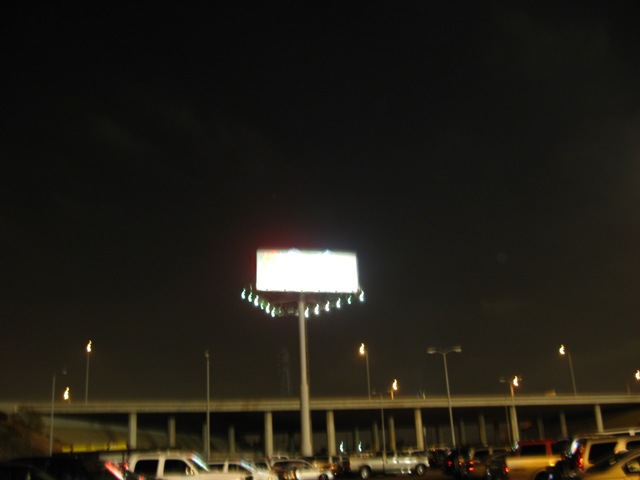The photograph captures a nighttime scene in a broad, rectangular format, featuring a parking lot illuminated by artificial lights. The sky is a deep, inky black, indicating it is well into the night. At the bottom of the image, several cars are neatly parked in at least two rows, all oriented to the right, suggesting an organized, possibly official parking area—potentially an airport parking lot.

In the middle-ground, there is an overpass stretching horizontally from left to right. This overpass doesn't cross any body of water, rather it serves as a bridge above the ground. Tall street lamps rise from the ground, casting their glow both over the parked cars and the overpass, contributing to the scene’s artificial lighting.

Dominating the upper portion of the scene is a very tall pole equipped with a triangular array of lights. Mounted on this pole, and facing directly towards the viewer, is a large billboard. The stark brightness of the billboard is such that no details or text are discernible, overshadowed by the intense illumination that obscures any potential message it carries. The overall contrast of the image accentuates the illuminated elements against the dark night, creating a dramatic juxtaposition between light and shadow.